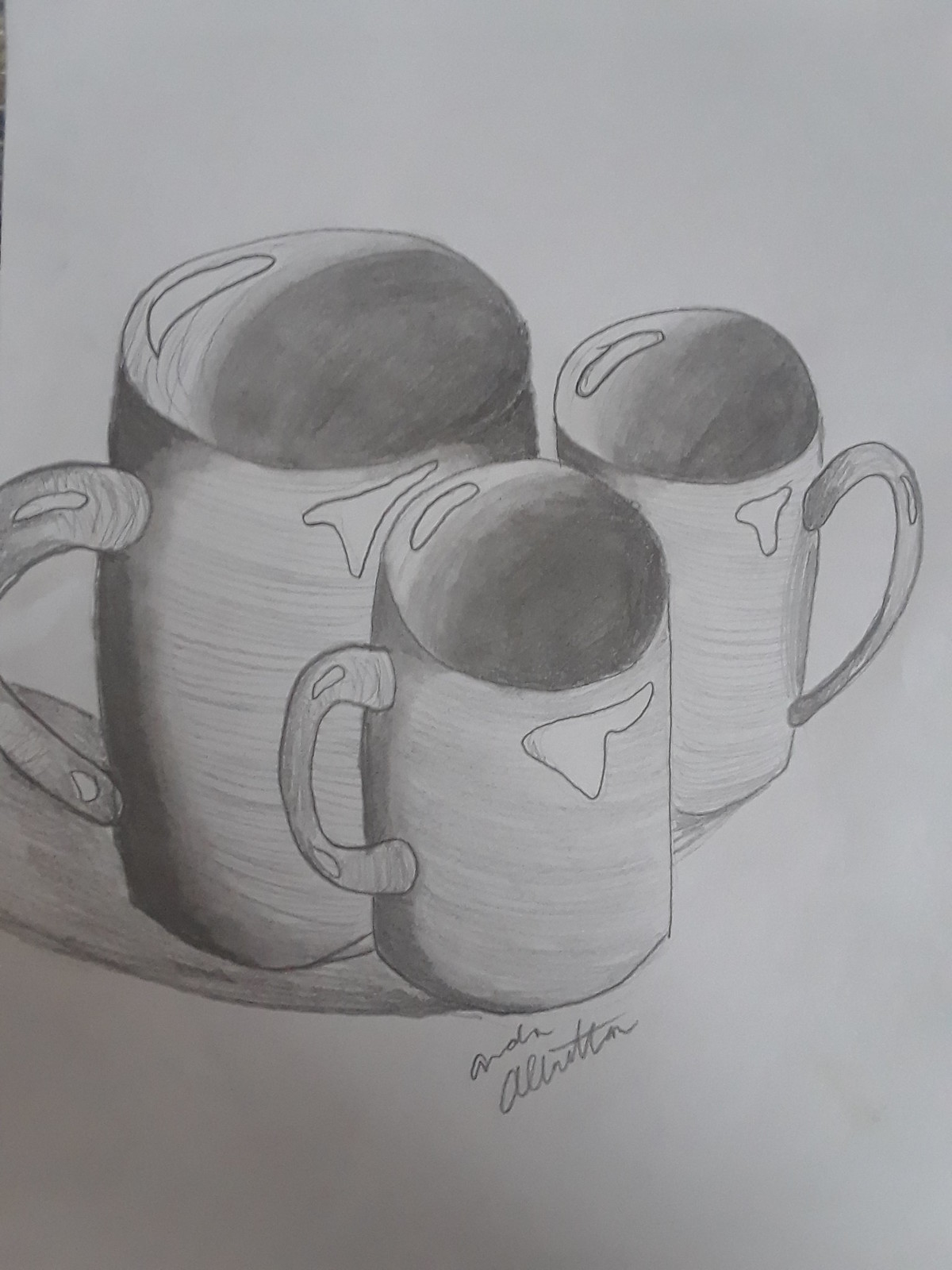This is a highly detailed pencil sketch depicting three coffee vessels viewed from a slightly elevated perspective, giving visibility into the interiors of the cups. The largest vessel, resembling a pitcher, sits on the left with its handle oriented to the left and features subtle shading and highlighted areas that suggest reflections. To its right are two smaller coffee cups with handles facing outward; their interiors are shaded darker to imply depth. The shading on both the interior and exterior of these cups creates a sense of light and shadow, adding to the realism of the drawing. The three vessels are positioned close to one another on what appears to be a white sheet of paper. At the bottom of the sketch, beneath the two smaller cups, there's an illegible signature, possibly reading "Andy Altraitor."